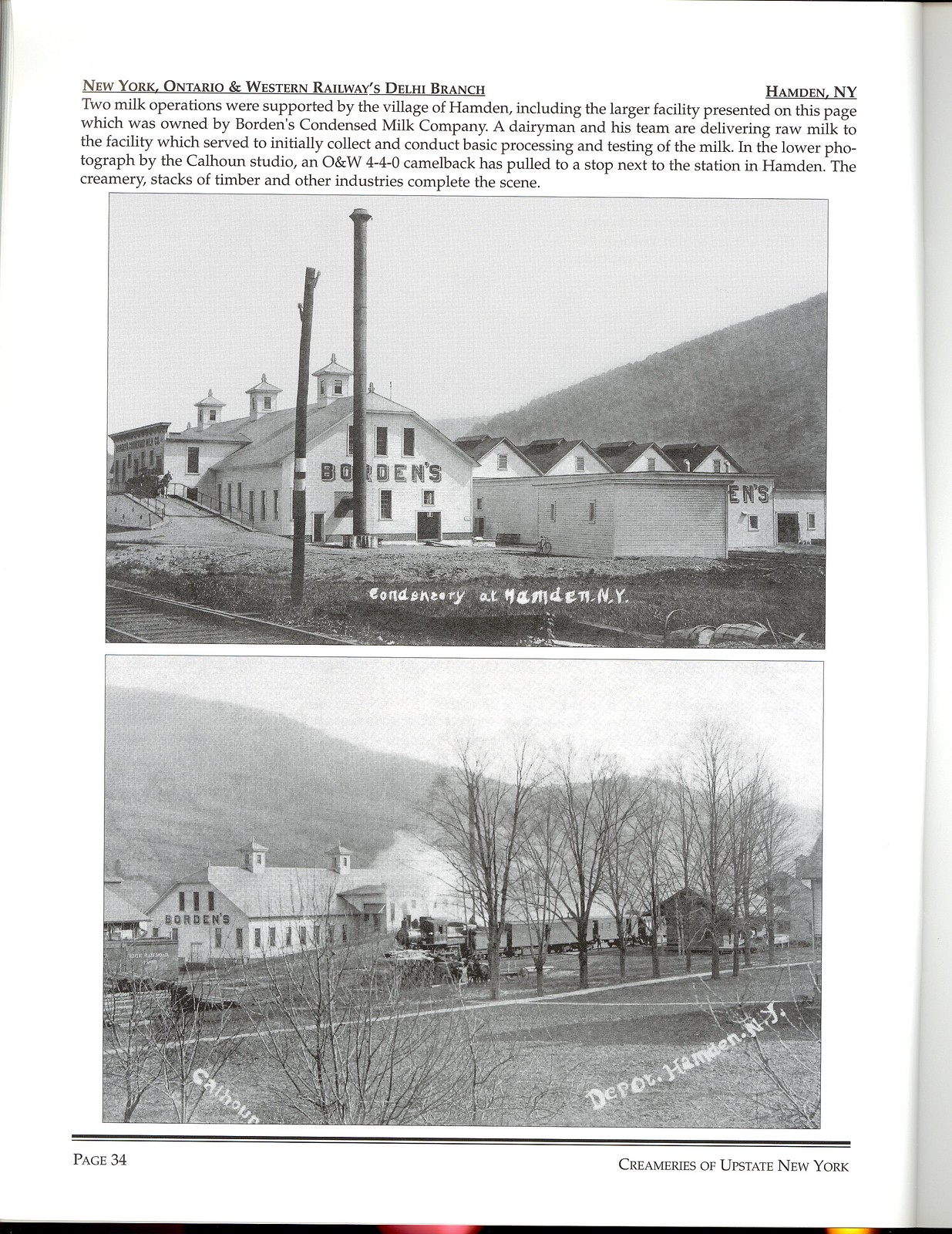The image depicts an open page from a book, specifically page 34, as indicated in the lower left corner. The top of the page carries the heading "New York, Ontario and Western Railways, Delta Branch" with a black line underneath, and "Hamden, New York" on the right. The central paragraph describes how two milk operations were supported by the village of Hamden, focusing on a facility owned by Borden's Condensed Milk Company. It details how a dairyman and his team deliver raw milk to this facility for initial collection, basic processing, and testing. 

The page features two black-and-white photographs. The top image depicts a white building with arched roofs and prominent tall columns with pointed tops. The front of the building clearly displays the name "Borden's," with the caption "Condoroy, Elmondrin, New York" beneath the picture. The lower photograph, credited to the Kowloon Studio, shows the same building from a different angle, facing left. The building has white walls, a pitched roof with pointed tops, and is flanked by bare trees on the left, with a rolling hill in the backdrop. In front of the building, an ONW 440-0 Camelback steam engine has stopped next to the Hamden station, complementing the industrious scene along with the creamery and stacks of timber. This photograph is captioned "Depot Hamden, New York" below it. The bottom right corner of the page states "Creameries of Upstate New York."